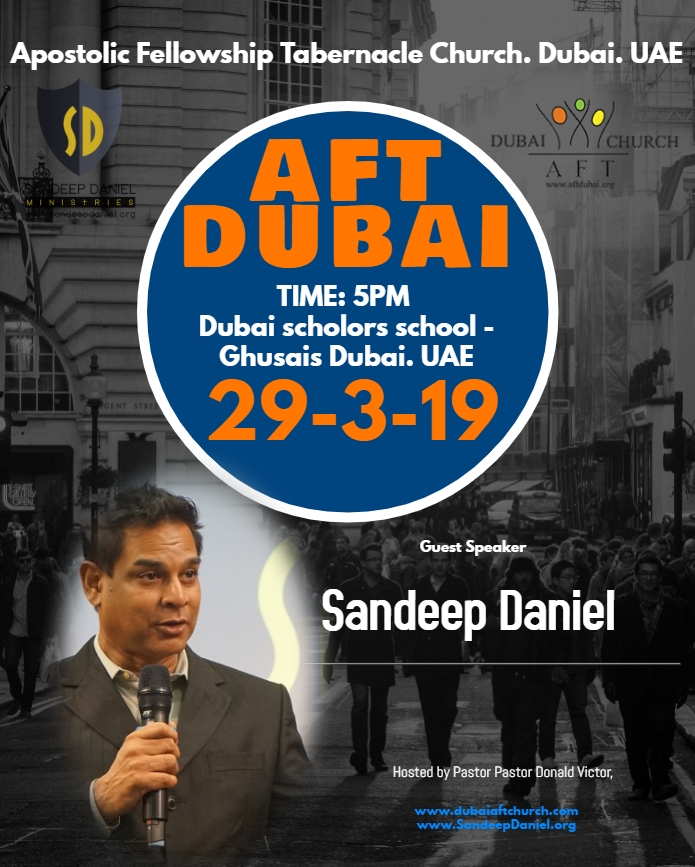This black-and-white image serves as an advertisement poster for the Apostolic Fellowship Tabernacle Church event in Dubai, UAE. The background features a lively street scene with people walking, cars passing by, and surrounding buildings. At the top of the poster, large white text reads "Apostolic Fellowship Tabernacle Church Dubai UAE," flanked by a grey shield logo with "SD" on the left and the Dubai Church AFT logo on the right. Dominating the center, there's a blue circle with a white outline and orange text that says "AFT Dubai." Beneath it, white text details the event time and location: "Time 5pm at Dubai Scholar's School, Ghusais, Dubai, UAE," with the date "29-3-19" in orange. Below, the poster announces the guest speaker in white text: "Sandeep Daniel." A white line separates this information from the host details at the bottom right, which states "hosted by Pastor Donald Victor." On the bottom left, there's a photo of the pastor holding a black microphone, characterized by his olive skin, short brown hair, a white shirt, and a brown jacket.